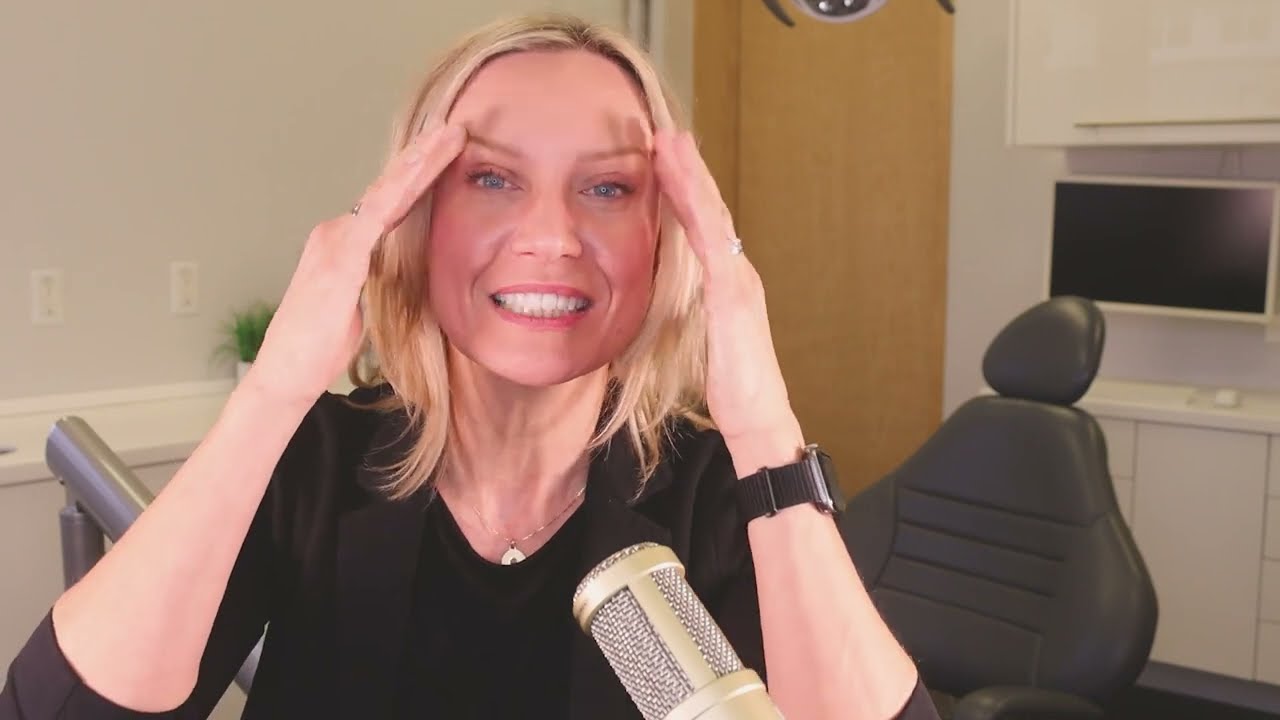In the image, there is a middle-aged woman with blonde hair cascading around her face, gazing directly at the camera and smiling warmly, revealing her gleaming white teeth. Her expressive blue-gray eyes are highlighted as she holds her hands up to her temples, almost as if she is playfully peering through them like binoculars. She wears a black long-sleeved shirt, slightly rolled up at the arms, paired with a black suit jacket. Around her neck is a silver necklace with a circular pendant, and an Apple Watch adorns her left wrist, complemented by a wedding ring.

In front of her is a tan and metal microphone, suggesting she might be in the midst of an interview or a podcast recording. The setting behind her resembles an office environment, featuring a black chair and a white wall. A computer screen can be seen behind the chair, and there is also a potted plant slightly obscured by her left hand. Additionally, the wall includes two electrical outlets, a brown door to the right, and a set of cabinets framing a TV screen mounted between them. The overall ambiance hints at a professional yet relaxed scene, possibly within a workspace or a dentist's office.